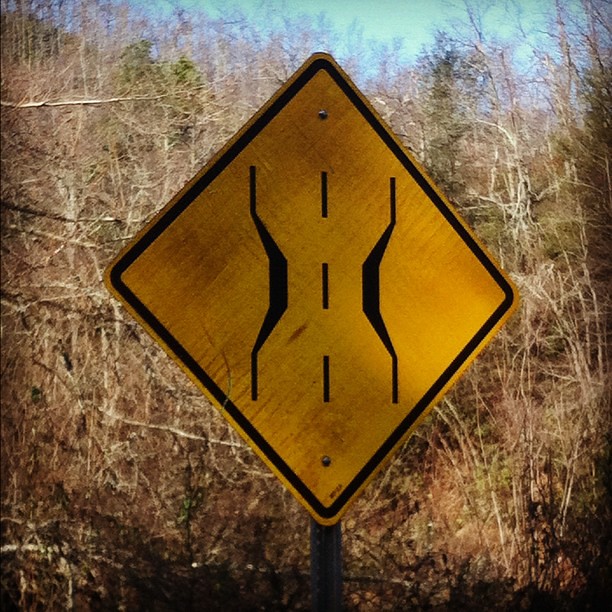The image features a yellow diamond-shaped traffic sign prominently displayed in the foreground. The sign contains a black graphic depicting the narrowing of the road, indicating that a narrow bridge lies ahead. Surrounding the sign, the background consists of a wooded area filled with barren trees, their leafless brown branches reaching skyward. A small patch of sky is visible above the treetops, adding a hint of openness to the otherwise dense woodland. The scene exudes a quiet, slightly desolate atmosphere, typical of a late autumn or early winter setting.